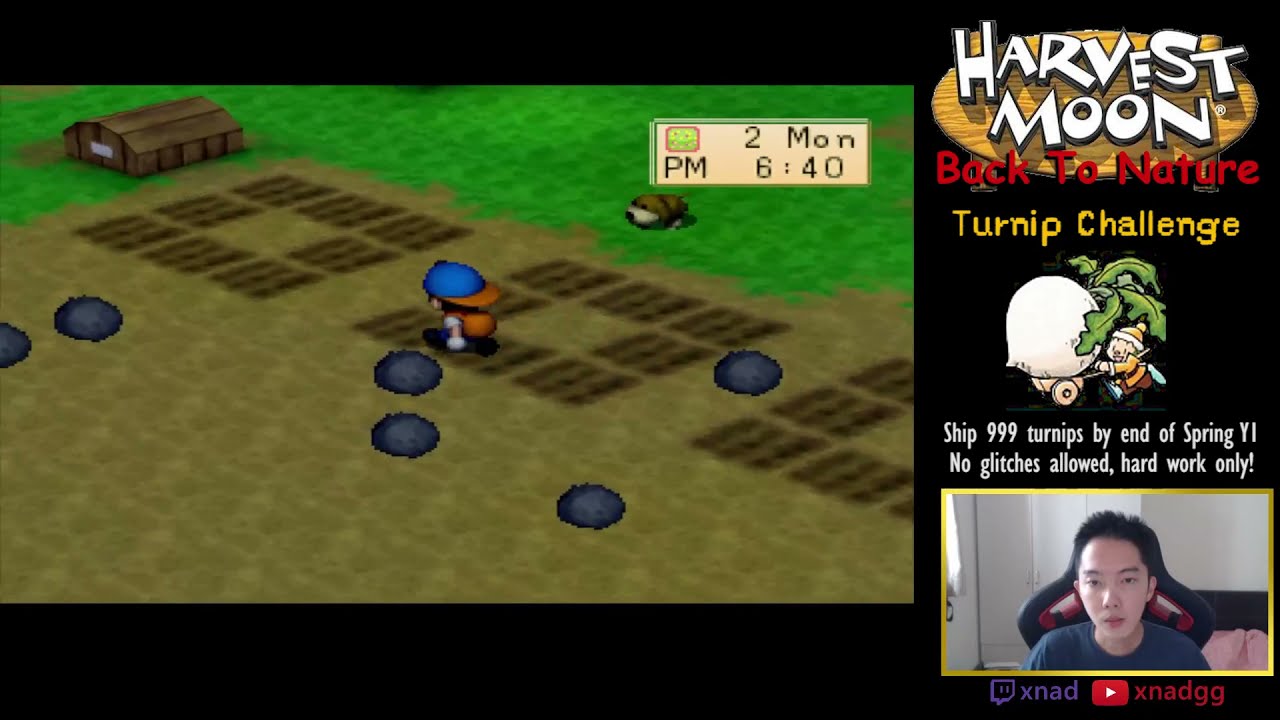The image is a detailed screenshot from a video game, specifically "Harvest Moon: Back to Nature," highlighting a turnip challenge. The game screen includes a green and brown landscape where a small character, resembling a farmer in a blue hat, is tending to his farm, which is partitioned by rocks. In the game, the challenge is to "Ship 999 Turnips by End of Spring Y1," which must be achieved with "No Glitches Allowed" and "Hard Work Only." On the right side of the screen, clear white letters outline the game's title and challenge details. Additionally, there's a blue-circled icon displayed on the screen. The lower right corner of the image shows an image of an Asian man in a gaming chair, deeply focused, wearing a blue shirt, depicted as the person playing the game. The surrounding area has a black background, with the labels "XNAD" and "XNADGG" visible near the bottom.